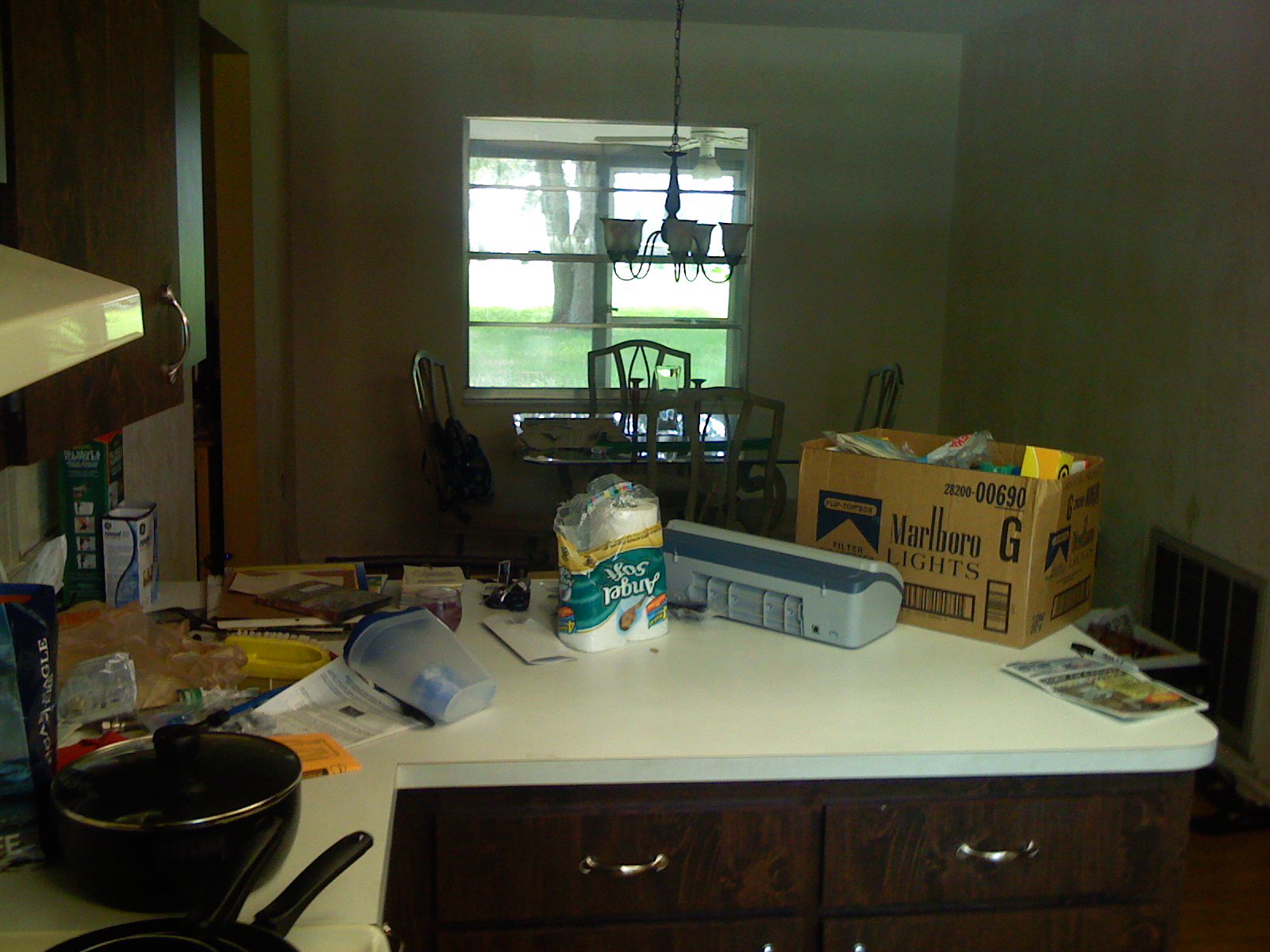The photograph captures a cluttered kitchen space looking towards a dining area. The white countertop is strewn with numerous items, creating a sense of disarray. Prominently, there is a four-pack of Angel Soft toilet tissue with one roll missing. A Tupperware pitcher with a lid, presumably used for storing juice, lies on its side among various scattered pieces of paper and a newspaper-style advertising circular. A device that appears to be either the back of a printer or a shredder adds to the clutter. Additionally, a large Marlboro Lights box, likely repurposed from a grocery store, sits prominently. Two pans are in sight: one resting on the counter near the stove, and another on the burner of the stove. The countertop itself is white, contrasting with the dark wood color of the drawers and cabinets that frame the kitchen.